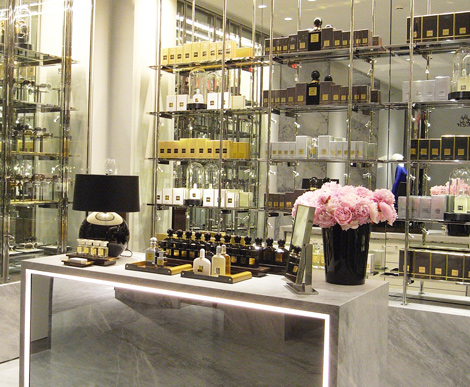The image depicts an upscale fragrance counter within a luxurious department store. Central to the scene is a sleek, gray marble table with matching marble sides, elegantly adorned with a black vase filled with pink peonies or carnations, adding a touch of vibrant color. The table is illuminated by a modern, black lamp, which echoes the hue of the perfume bottles neatly arranged in front. Surrounding this central feature, there are vast silver shelves holding a variety of meticulously arranged fragrance boxes in shades of white, black, beige, gold, and brown, each suggesting an exclusive range. Behind these shelves, the reflection in a mirror further amplifies the opulence and spaciousness of the department, emphasizing the absence of any shoppers or staff, indicating a quiet moment in this refined retail space.